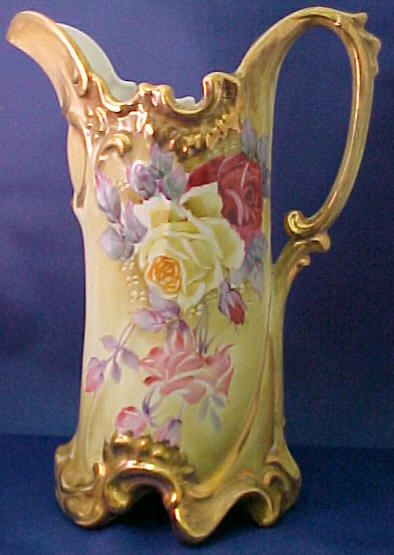The image showcases a highly ornate water pitcher, which could also double as a vase due to its elaborate design. The pitcher features a sweeping handle and a long pouring spout, both in a luminous golden-yellow hue that extends around the top, down the side, and around the base. The upper part, handle, and mouth brim with gold detailing. The main body of the pitcher is adorned with an intricate floral pattern, featuring prominently painted roses in red and yellow, accompanied by violet, pink, and smaller rose buds, all meticulously hand-painted. The background presents a clean and simple setting with a blue wall and a white or blue surface, emphasizing the vivid details and craftsmanship of the pitcher without any distracting context or other objects.